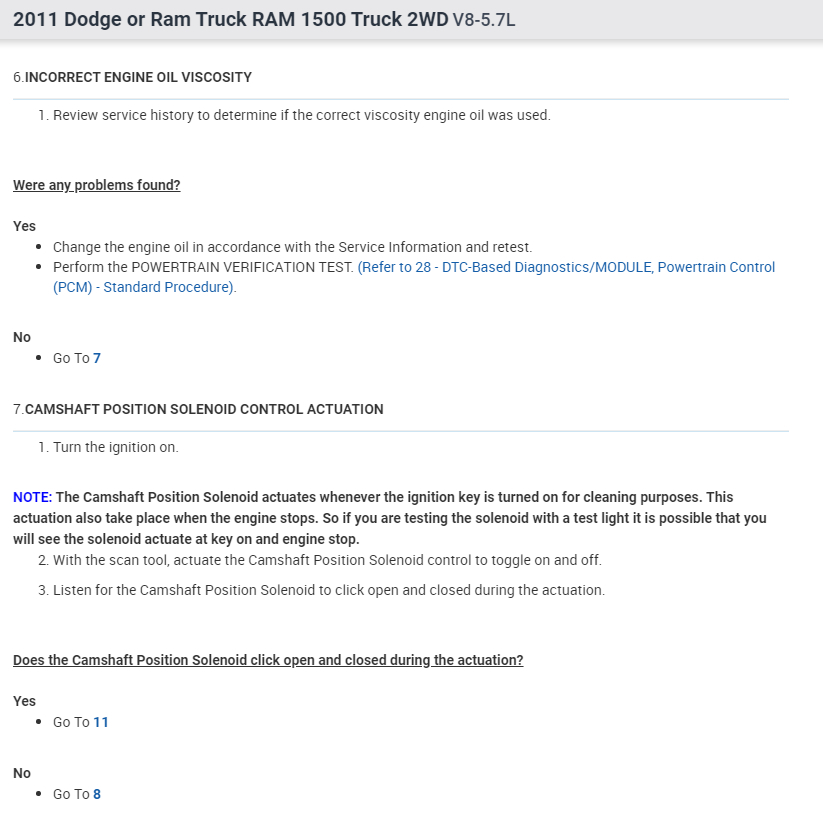**Detailed Caption for Screenshot:**

The screenshot appears to be an enlarged capture from a smartphone. It details troubleshooting steps for a 2011 Dodge RAM 1500 truck, specifically a 2-wheel drive model with a V8, 5.7-liter engine. The diagnostic process begins at step number 6 with a note on incorrect engine oil viscosity. The first step advises reviewing the service history to check if the correct engine oil viscosity was used.

The next part is a question asking if any problems were found, followed by a "Yes" answer. Two actionable bullet points are listed:
1. Change the engine oil according to the service information and retest.
2. Perform the powertrain verification test.

If no problems were found, the instruction is to proceed to step 7, which focuses on the camshaft position solenoid control actuation.

Step 7 includes:
1. Turning the engine on, accompanied by a note explaining that the camshaft position solenoid actuates when the ignition key is turned on for cleaning purposes and also when the engine stops. Therefore, when testing the solenoid with a test light, the actuation could be observed at key-on and engine stop.
2. Using a scan tool to toggle the camshaft position solenoid control on and off.
3. Listening for the solenoid to click open and close during the actuation.

The subsequent question asks if the camshaft position solenoid clicks open and close during actuation. If the answer is "Yes," the next step is to proceed to step 11. If "No," the direction is to move to step 8.